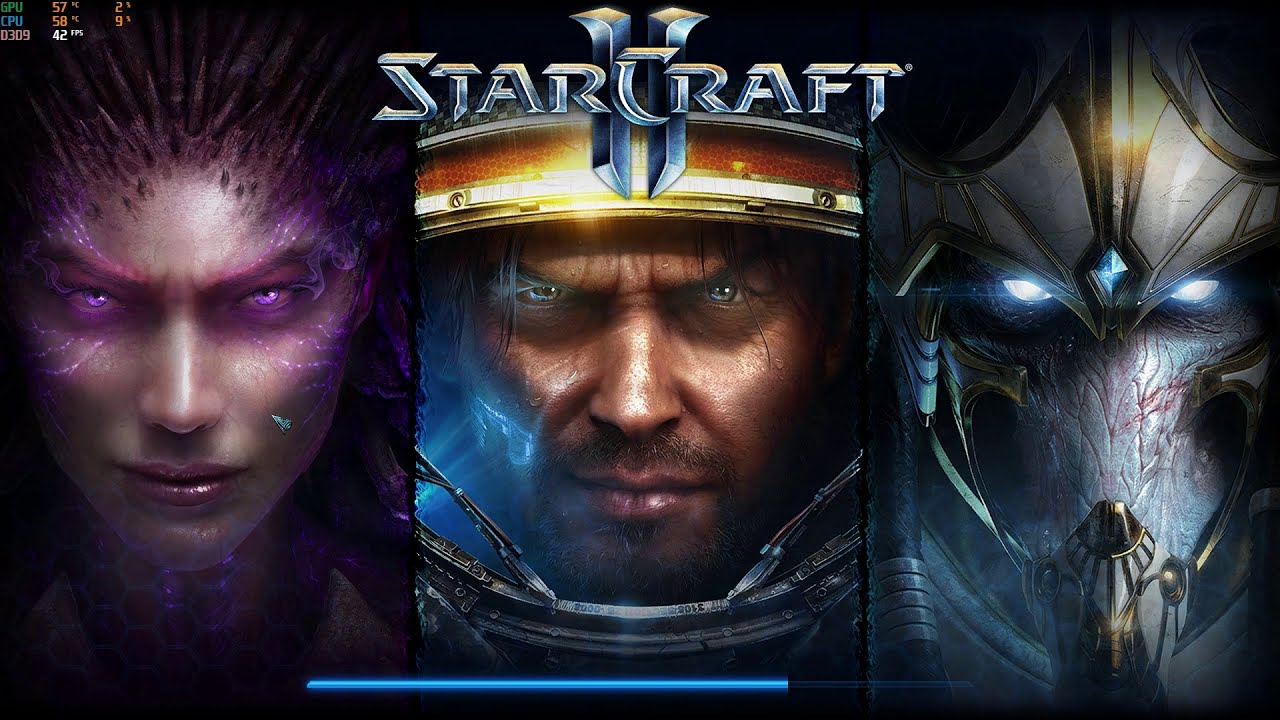This image appears to be the cover art for a science fiction video game, titled "Starcraft 2", prominently displayed in silver text at the top center. The image is divided into three equal segments, each featuring a distinct character. 

On the left, there is a fierce-looking female character with violet eyes, and violet veins extending toward her cheekbones. Her hair is uniquely styled into demonic spikes. 

In the center, we see a man with blue eyes, brown hair, and stubble, wearing an astronaut-like helmet adorned with LEDs across the forehead and featuring small windshield wipers on the rim.

The right segment showcases an alien or machine-like figure with glowing blue, diamond-shaped eyes, and a forehead marked with a diamond symbol. He is distinguished by a helmet that resembles Roman imperial design and has dreadlock-like features.

The background and color palette include shades of tan, brown, purple, light blue, orange, blue, gray, and yellow, evoking a science fiction ambiance typical of a game cover for console or PC.